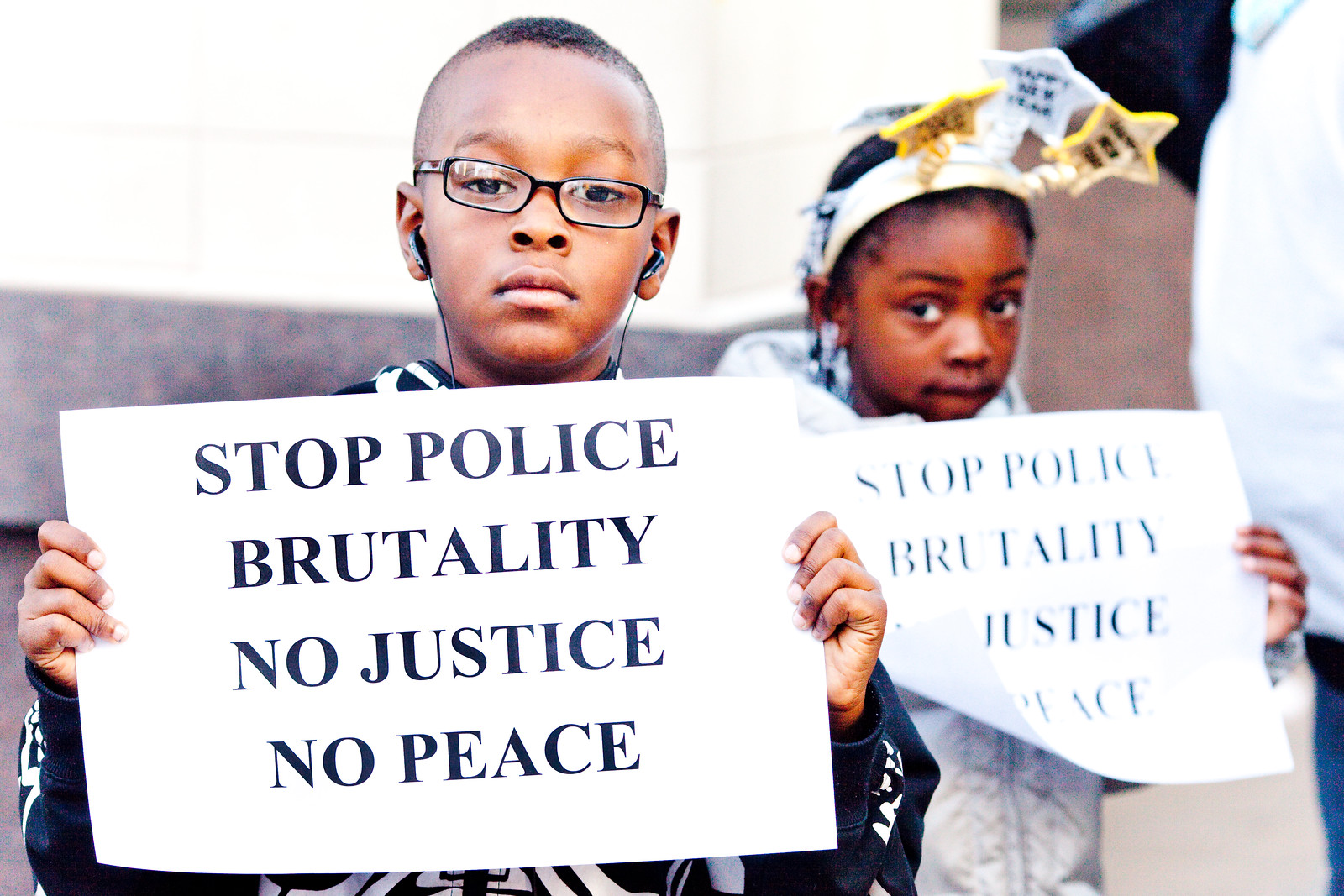This is a photograph capturing a moment of protest featuring two young Black children, a boy and a girl, both holding signs. The boy on the left, looking serious and studious, is wearing sunglasses and earphones. He holds a white sign with blue text that reads, "Stop Police Brutality, No Justice, No Peace." To his right stands a younger girl, wearing a hat and a white coat, also holding a sign with the same message. She sports a headband adorned with three large stars. An adult figure is partially visible on the right, though their face is not shown. In the background, a white building is discernible, adding context to the protest setting.